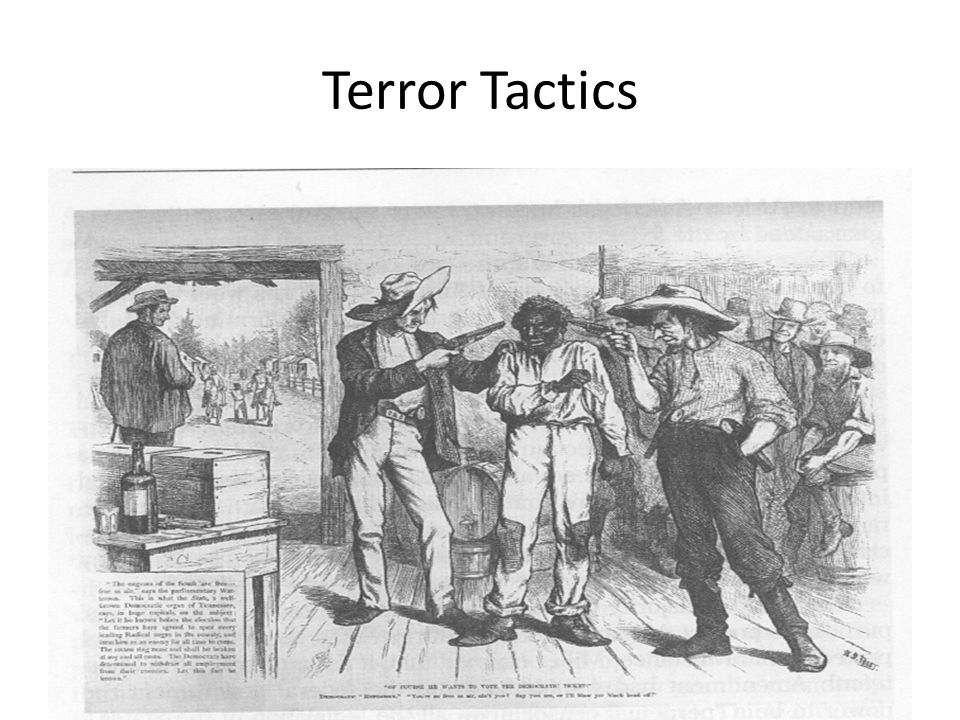The image is a black-and-white illustration, likely a printout or a screenshot from a historical textbook or magazine. At the top, there is a white banner with the bold, capitalized text "TERROR TACTICS." The illustration below, drawn in pencil, depicts a tense and distressing scene from an older time, evocative of the era of slavery or the Old West. 

At the center of the drawing, an African-American man is surrounded by several white men, all of whom are wearing cowboy hats. Two of these men stand close to him, each holding a gun pointed at his head. One of them has his head facing downward, while the other has one hand in his pocket. The African-American man appears fearful, with one arm raised and the other down by his side, glancing off to the right. 

In the background, more white men, possibly cowboys, look on with apparent interest. The setting includes a wooden plank floor, kegs scattered around, and a table with a bottle of liquor. To the left side of the image, there is an entrance or doorway with another man standing, back facing the viewer and partially looking over his shoulder. Outside the doorway, there seem to be horses and potentially another enslaved person. At the bottom of the illustration, there is text, although it is too small to read clearly, along with a square black box containing a paragraph. The overall composition of the image heavily centers the distressing scene at the bottom with the stark title above, contributing to its educational and historical impression.